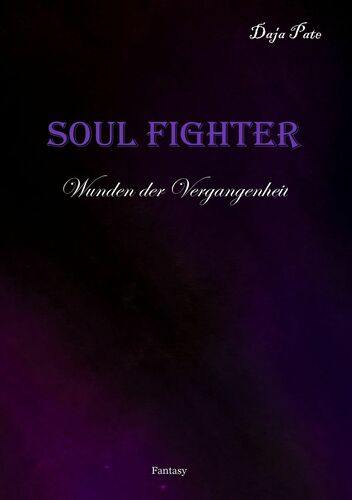The image is a rectangular book cover with a swirling gradient background of purple and black hues. The gradient transitions from lighter shades of purple and pink at the bottom to darker purples and blacks towards the center, then gradually back to a regular purple. At the top of the cover, in a delicate white script font, are the words "Daja Pate." Below this, the book's title "SOULFIGHTER" is prominently displayed in uppercase purple letters. Beneath the title, another line in the same white script font reads "Wunden der Vergangenheit," a German phrase. At the very bottom, "Fantasy" is written in a small, white, Times New Roman-like font.